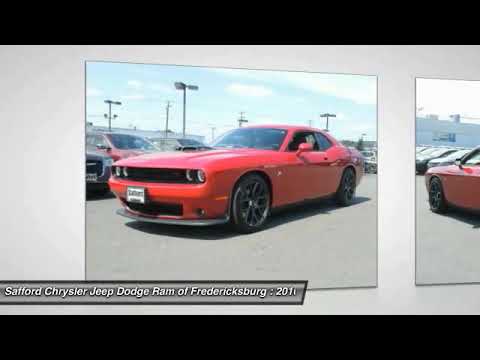The image displays a detailed, angled view of an older red Chrysler, possibly a Dodge Challenger, prominently featured with two near-identical pictures of the car. The main picture shows the car facing slightly left, revealing the driver's side window, side panel, black tires, and an inset black front grille. Behind the car, other vehicles, light posts, and a pale gray surface are visible. To the right, a cropped, mirrored image of the car facing right complements the main picture. Both images appear on a white background set at a diagonal angle. The image is framed by thick black horizontal bars at the top and bottom. At the bottom left corner, a silver box with a dark gray outline contains the text "Safford Chrysler Jeep Dodge Ram of Fredericksburg" in white font, with the partially visible number "2011." The overall scene is in natural daylight with blue skies and white clouds, hinting at a car dealership advertisement.